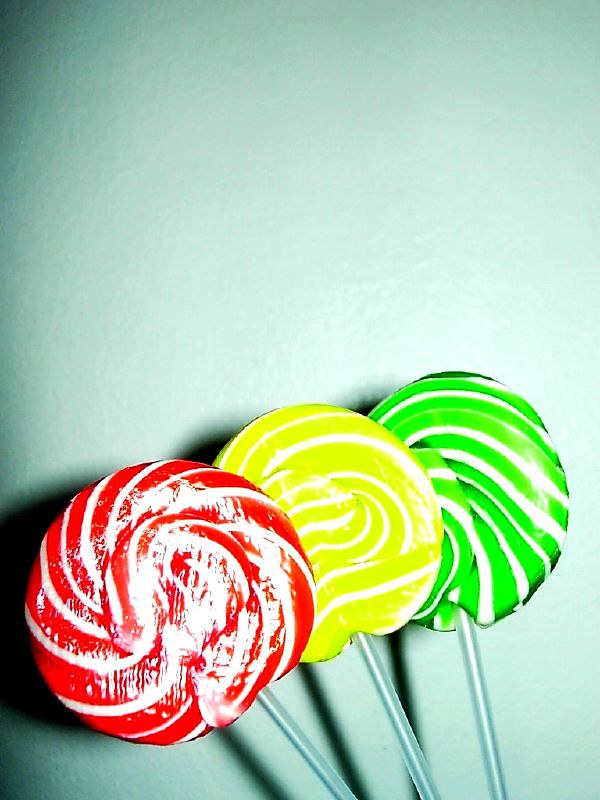In the color photo, three hard candy lollipops are prominently displayed, each attached to a white or clear stick. The lollipops exhibit swirled patterns in distinct colors: the one on the left features red and white swirls, the middle lollipop has yellow and white swirls, and the one on the right displays green and white swirls. These vibrant candies are arranged in an overlapping manner, with the red lollipop positioned in the front, followed by the yellow and then the green. They cast a shadow against a textured light blue-green background, creating an eye-catching contrast. The lollipops have a glossy finish, enhancing their shiny appearance. The surrounding area beneath them transitions from a brighter white to a darker, almost greenish hue, depending on the light's reach. The absence of people or text keeps the focus entirely on the colorful lollipops, suggesting they might be cherry, lemon, or apple/lime flavored.